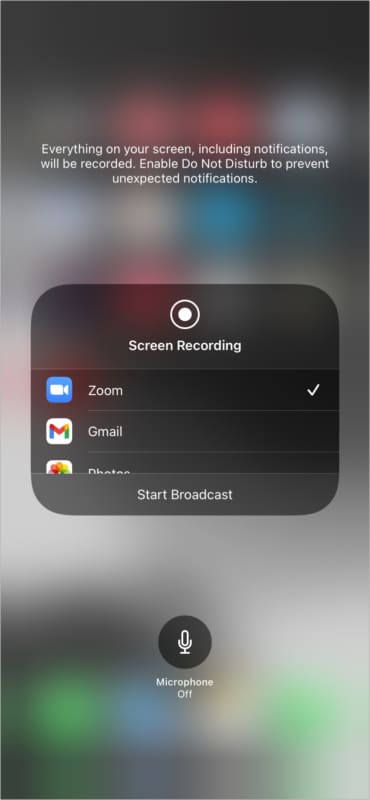This image depicts a screen overlay under the "Websites" category, which is providing a message about screen recording. The message alerts the user that everything on their screen, including notifications, will be recorded and advises enabling "Do Not Disturb" to avoid unexpected notifications. The message also references "Screen Recording," with Zoom already selected. Below Zoom, Gmail is listed, and there appears to be another app, but its identity is obscured. The overlay includes options such as "Start Broadcast" and shows that the microphone is turned off.

In the blurred background, a variety of app icons are visible in different colors—red, blue, green, and white—indicating a cluttered home screen filled with numerous applications. However, the specifics of these icons are not clear, and no details are provided that reveal the type of phone or the time of day. The image gives the impression that the user is preparing to start a Zoom call or a screen recording session.